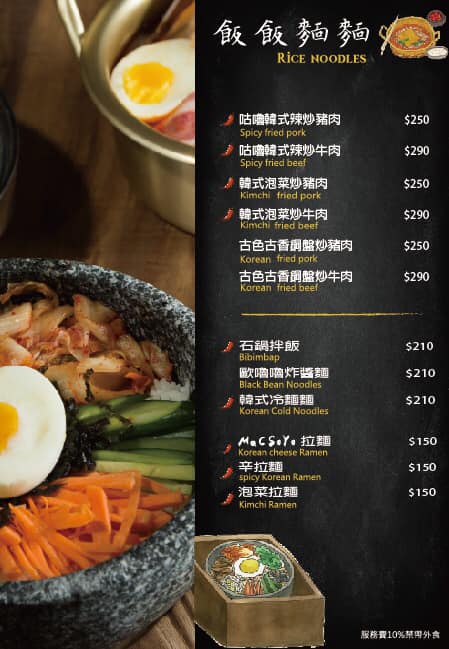This image showcases a detailed menu for what appears to be a Chinese restaurant with a strong Korean cuisine influence. The menu prominently features white text in Chinese characters on a black background, with English translations and pronunciations provided underneath. The menu includes a variety of dishes, such as rice noodles (the only English heading on the menu), spicy fried pork ($2.50), spicy fried beef ($2.90), kimchi fried pork ($2.50), kimchi fried beef ($2.90), Korean fried pork ($2.50), Korean fried beef ($2.90), bibimbap ($2.10), black bean noodles ($2.10), Korean cold noodles ($2.10), Korean Chinese ramen ($1.50), spicy Korean ramen ($1.50), and kimchi ramen ($1.50). Spicy dishes are marked with a small red pepper graphic to indicate their heat level. To the left of the text, there are illustrative images of some of these traditional Korean dishes, including one in a stone pot containing carrots, cucumber, and an egg atop rice. Additionally, there is a drawing of a dish within a box on the bottom part of the menu, adding a hand-drawn, artistic element to the presentation.